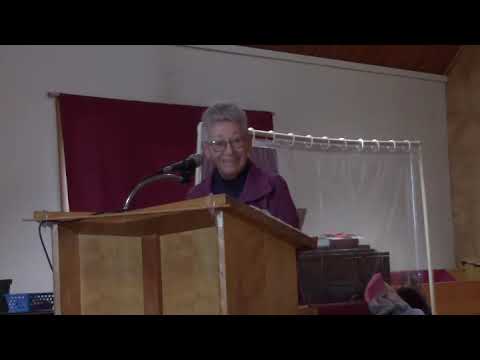In the image, an elderly woman is standing at a wide podium, smiling towards the camera. She's wearing wide round-frame glasses, a purple leather jacket over a collared dark blue or dark purple shirt, and has short gray hair. A silver microphone is extended towards her face. The backdrop features a room with a white wall and a window adorned with a maroon or dark red curtain. Above the window, a translucent curtain with shower curtain rings is draped from a silver pole. Additionally, the right side of the image reveals a brown wooden wall and a glimpse of a brown wooden ceiling. Behind the sheer curtain, a table or some furniture is partially visible through the transparent fabric.